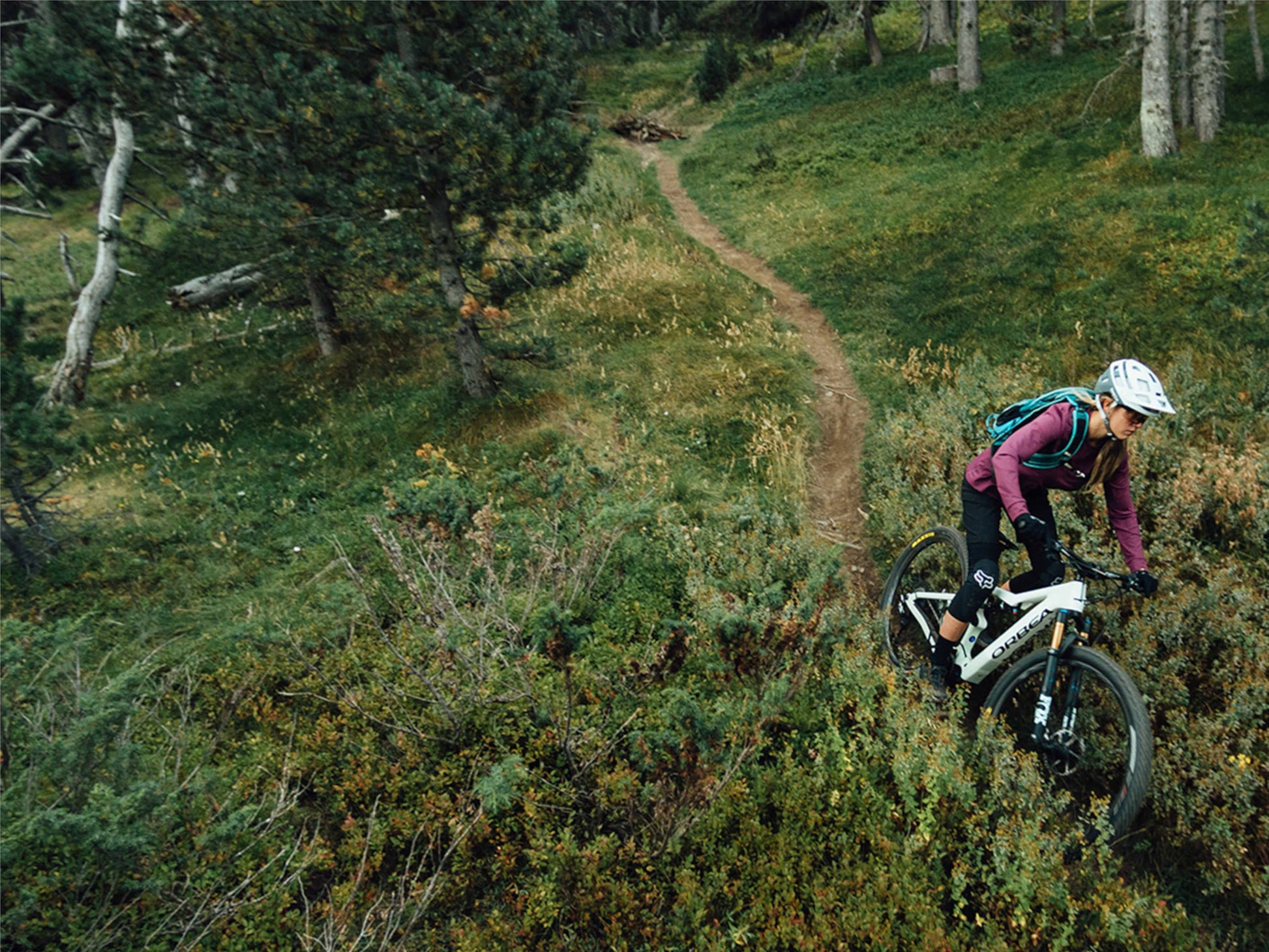A woman rides a mountain bike along a narrow dirt trail through a rugged, natural landscape. Clad in a purple long-sleeved thin sweater, tight leggings, black shoes, and a white helmet, she is poised on her white-framed bike with black tires. A teal backpack rests on her back, and she wears gloves for grip. The terrain is characterized by dark green grass and dense, unkempt bushes on either side of the trail. The scene is dotted with tree trunks—some ash white-gray and others darker with pine-like foliage—interspersed with brush, sticks, and patches of dead grass. The photograph is taken from an elevated angle, looking down on the cyclist as she navigates the wild, untamed environment.